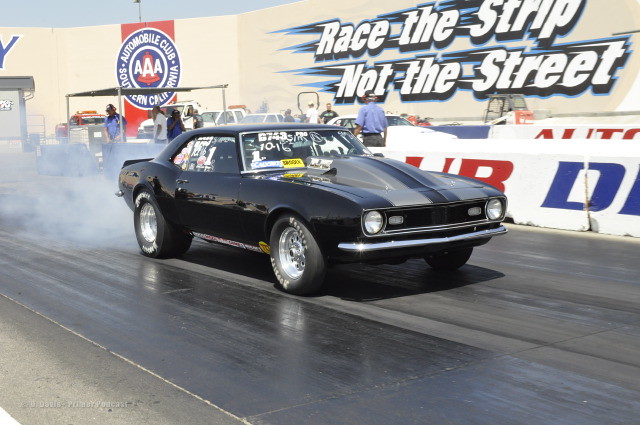In this detailed image, a sleek black muscle car, designed for racing, dominates the scene. The car features white lettering on its windshield and side windows, gray accents on the hood, and a prominent hood scoop, suggesting high performance. The setting is a race track that stretches diagonally from the bottom left to the top right of the image. Behind the car, there's a noticeable tan-colored raceway wall with an italicized white slogan, "Race the Strip, Not the Street," enhanced by streaks of black and blue. To the left of the sign, a tent area can be seen along with people gathered near various signs, adding to the lively atmosphere. Further into the background are ordinary cars and trucks, contrasting with the racing scene in the foreground. A plume of smoke rises behind the car, indicating recent high-speed action. The top left corner reveals a small patch of sky, confirming that it's a daytime event under clear conditions. The left section of the image also has the text, "Automobile Club AAA, Southern California," highlighting the involvement of the well-known automotive organization in the event.